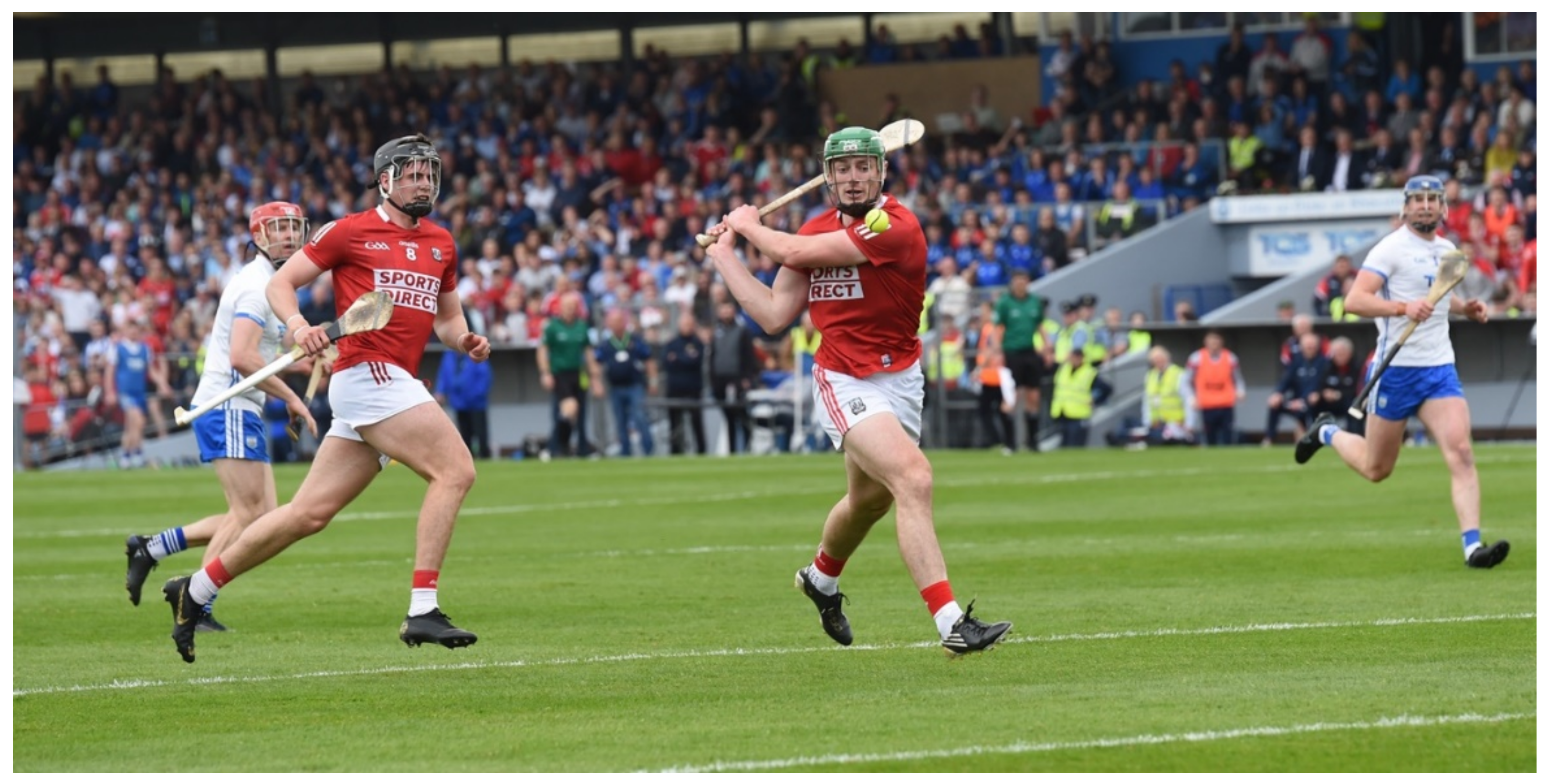This outdoor daytime photograph captures an intense moment during what appears to be a hurling match, although some might confuse it with cricket or lacrosse. The rectangular image, roughly five to six inches wide and three inches high, is dominated in the lower half by a lush green field marked with thin horizontal lines. Above the field, a stadium filled with spectators in colorful attire watches intently from the bleachers.

On the field, four athletic men of Caucasian descent are mid-action: two teams, each comprising two players. The central figures wear red short-sleeved shirts paired with white pants, black cleats, and helmets with face masks. Their competitors on the periphery sport white short-sleeved shirts with blue shorts and black cleats, also donning protective helmets. Each player wields a large stick used in the game. The player at the front center is dramatically posed with his stick raised over his head, seemingly in the act of hitting a small yellow ball that hovers in the air near his face, capturing the dynamism of motion as three of the four players appear slightly off the ground. This action-packed scene suggests a snapshot of a fierce two-on-two competitive play, set against the backdrop of enthusiastic fans.